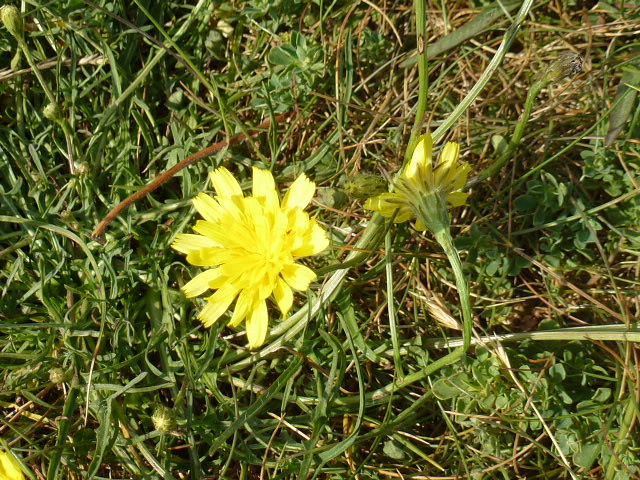In this bright, top-down photograph of a grassy area, two small, solid yellow flowers are prominently featured. The grass appears tall, somewhat messy, and intermixed with weeds and four-leaf clovers, suggesting it hasn't been mowed for a while. The flower in the center-left is fully bloomed with its dense yellow petals fanned out, resembling a small dandelion. To the right, another flower lies flat on the ground, as if trampled, revealing its green stem and underside of the petals. In the very bottom left corner, a yellow petal peeks into the frame, hinting at yet another flower. The entire scene appears lively and untamed, basking in the brightness of the day.